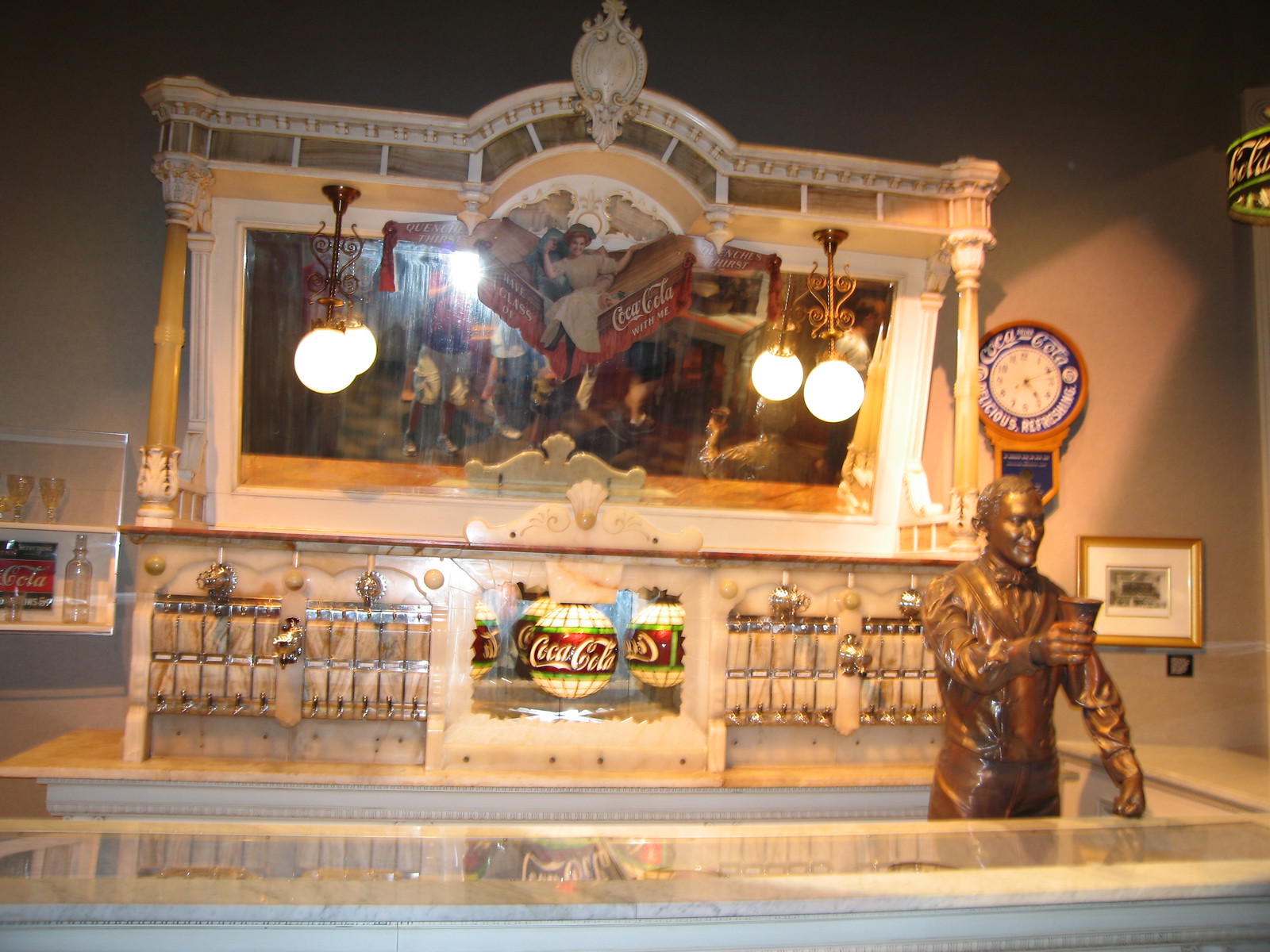This image captures the ornate and historical charm of what appears to be a mock-up of an old-fashioned bar, likely within a Coca-Cola museum or an Americana exhibit. The centerpiece is a large, rectangular mirror adorned with intricate designs, including a figure of a woman on top and flanked by two Corinthian columns, creating a castle-like architectural impression. Hanging above the mirror are two ball-shaped lights that illuminate the scene. Below the mirror, a counter with glass at its center displays various Coca-Cola memorabilia, including multiple glass bottles. 

Prominently featured behind the counter is a lit-up globe that reads "Coca-Cola," encased in an elaborate marble frame. To the right of this globe stands a bronze statue of a bartender, arm extended as if offering a drink. The statue introduces an element of nostalgia, suggesting the bar setting could be from the 1800s. Additional details like small drink-dispensing taps and a signage piece encroaching from the right with the word "Cola" contribute to the overall vintage feel. The entire scene is bathed in warm lighting that highlights the antique, yet pristinely maintained, aesthetic.